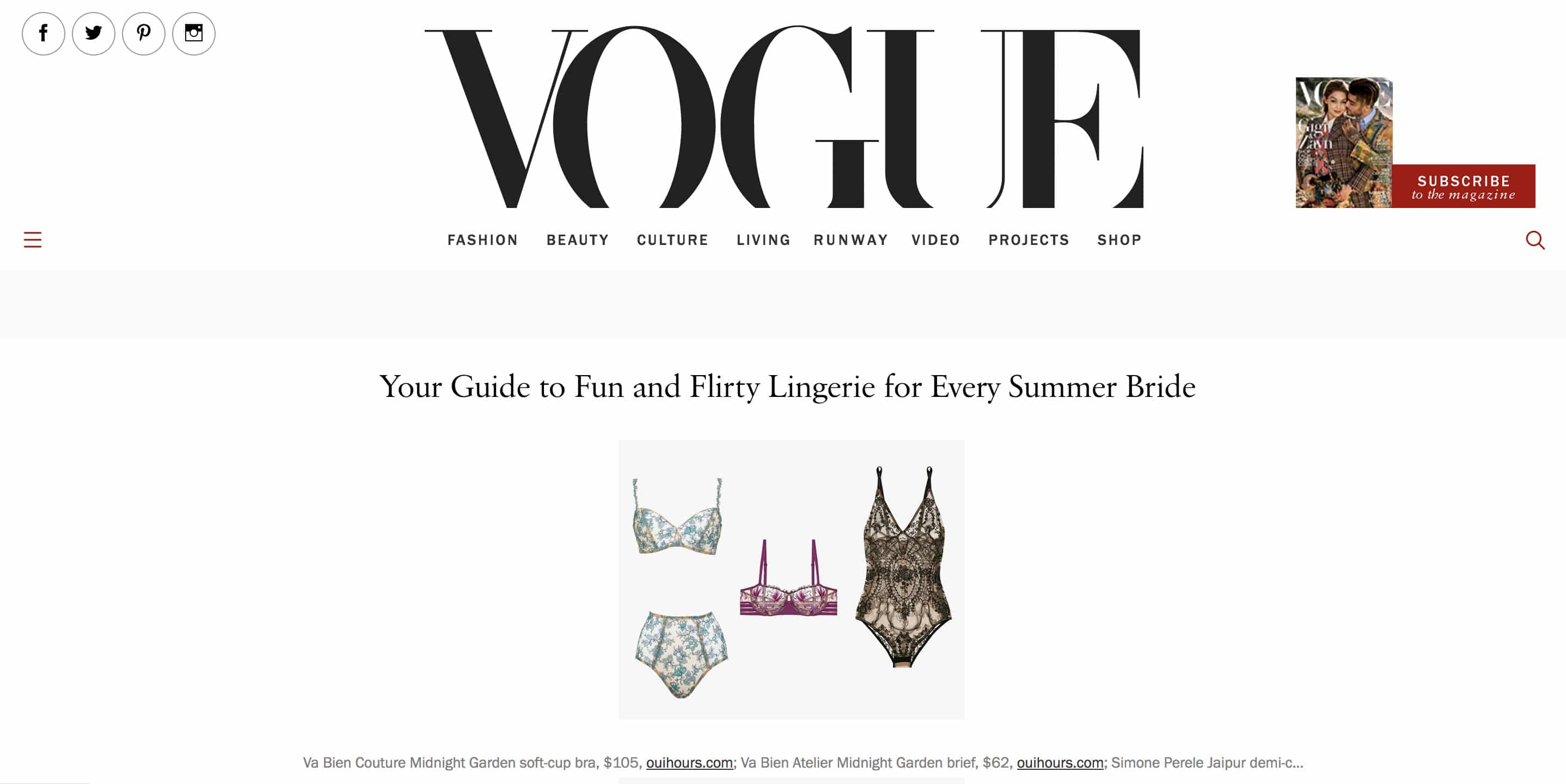This image appears to be from a website with a white backdrop. In the upper left-hand corner, there are several social media icons arranged horizontally: a white circle outlined in gray with a black "F" representing Facebook, followed by a white circle outlined in gray with a black bird icon symbolizing Twitter, and next, a white circle with a black "P" for Pinterest. Adjacent to these, there's a gray circle containing a small black box wearing black sunglasses—it's unclear what this logo represents.

Moving to the center of the page, there's a prominent "Vogue" logo, approximately two inches thick, in black text. Below the logo, the words "fashion," "beauty," "culture," "living," "runway," "video," "projects," and "shop" appear, all in black text. 

To the right of the page, there's an image taken from Vogue magazine showcasing the cover of their latest issue. This cover features a man and a woman portrayed as a couple, with the woman on the left facing the camera and the man behind her, leaning around and gazing at her affectionately. In the bottom right-hand corner of this magazine cover, there's a small section that says "subscribe" in white text.

Centrally, a headline reads, "Your Guide to Fun and Flirty Lingerie for Every Summer Bride." Below this headline, there are images of three different lingerie sets. The first set on the left is a white and blue floral bra and panty combination, with high-waisted panties. The middle set is a maroon and white-colored bra with a floral pattern. On the right, there is a beige one-piece bodysuit with black lace overlay and thin spaghetti straps.

Below these images, a line of text describes the items, but parts of it are blurred and difficult to read. It seems to mention "VIN Couture Midnight Garden Soft Cut Bra, $105" and "VIN Pacifier Midnight Garden Brief, $62," followed by a partially obscured web address. The rest of the text is too blurred to decipher.